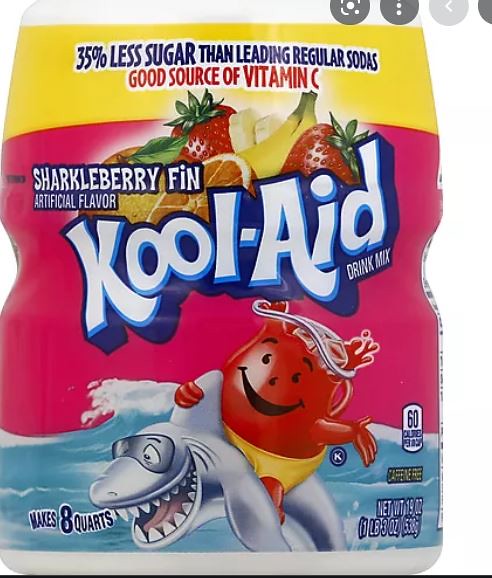This photograph showcases a plastic Kool-Aid container set against a completely white background. The container itself is white and prominently features a vibrant, colorful label. At the top of the label, a bright yellow band displays the text "35% less sugar than leading regular sodas" and "Good source of Vitamin C." Below this, a thicker pink band bears the iconic Kool-Aid logo in bold white letters. 

Further down, a blue band adorned with wave patterns frames a playful scene: a shark wearing goggles and a Kool-Aid jug character sporting yellow swim trunks. Above the pink band, an assortment of fruit suggests the beverage's fruity flavor, identified as "Charcoal Berry Fin - Artificial Flavor." 

In the bottom left corner of the container, it states that the mix makes 8 quarts. The bottom right corner includes details such as the net weight and asserts that the product is caffeine-free.